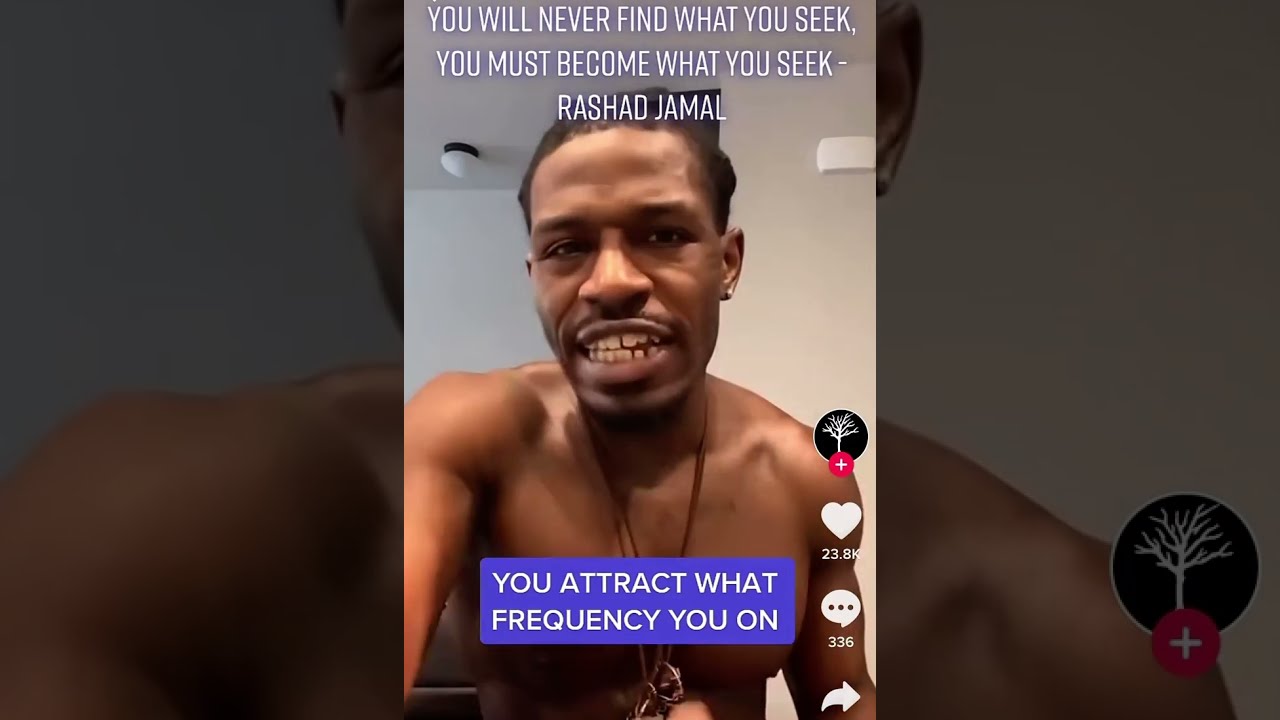This is a social media screenshot from either Instagram or TikTok featuring Rashad Jamal, a black man standing bare-chested in a white room with lights hanging from the ceiling. He looks straight into the camera, and the image is partially overlaid on a larger, slightly tinted black background of the same video. Rashad Jamal wears a large metal necklace around his neck. At the top of the screen, white text reads, "You will never find what you seek. You must become what you seek," attributed to Rashad Jamal. Across his chest, white letters on a blue rectangle state, "You attract what frequency you're on." To the right of the image, various social media icons are visible: a black circle with a white tree, a red circle with a plus sign, a heart icon with "23.8K" likes, a comment bubble icon with "336" comments, and a curved arrow.